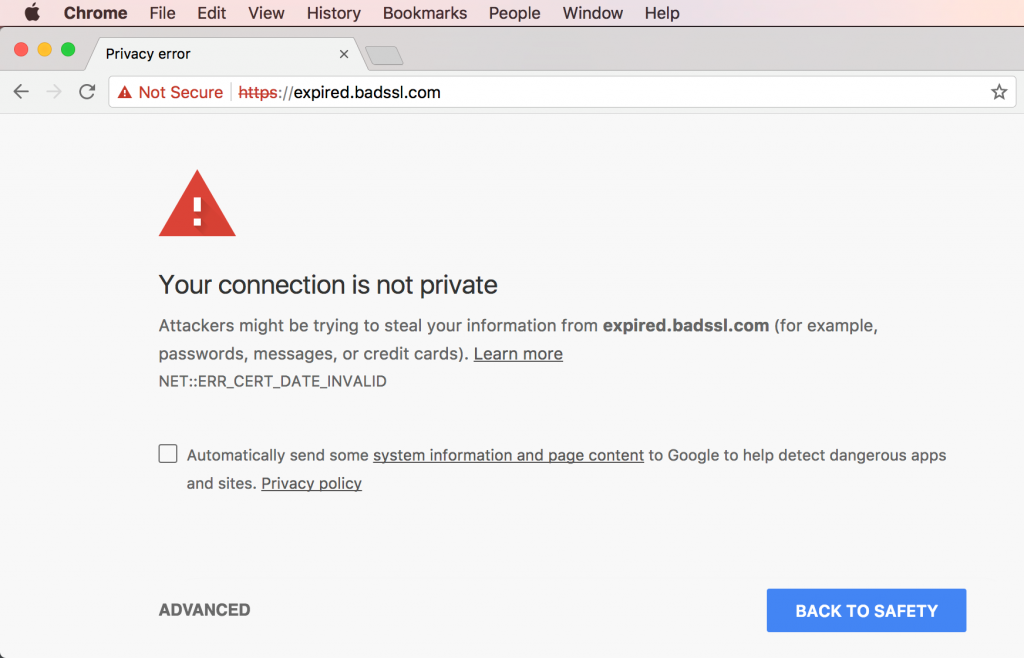Screenshot of a Google Chrome browser window on an Apple computer. The browser is displaying a warning page with the URL "expired-bad-ssi.com" in the address bar, which indicates possible security issues with the website. At the top, the browser displays a "Not Secure" warning along with a red triangle alert icon. The page features a prominent message that reads, "Your connection is not private," followed by an alert stating, "Attackers might be trying to steal your information from expired-bad-ssi.com." The alert specifically mentions that the information at risk could include passwords, messages, or credit cards, offering a "Learn More" link for further details. The typical Google Chrome menu options are visible at the top, including File, Edit, View, History, Bookmarks, People, Window, and Help, emphasizing that the screenshot was taken on a macOS interface.